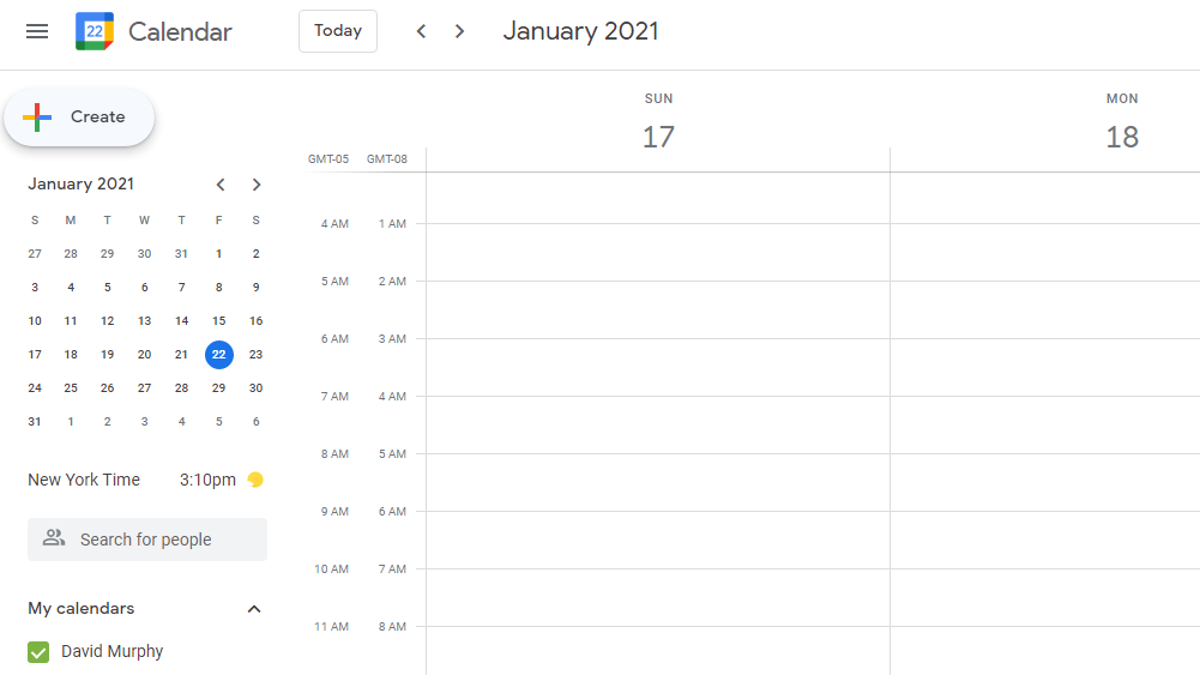This is a cropped screenshot of a Google Calendar interface, specifically displaying the date January 17, 2021. At the top left corner of the image, there is a recognizable Google Calendar icon. Adjacent to it, three labels are visible in sequence: "Today," "January," and "2021." Below these, on the left-hand side, a blue oval icon labeled "Create" is prominently displayed. Directly underneath the "Create" button, there is a mini monthly calendar showing the entire month of January, with the 22nd highlighted in blue.

Further down, it lists the current time zone as "New York time," accompanied by a grey "Search for people" button. At the bottom of this panel, the "My calendars" section is expanded, revealing a calendar named "David Murphy," which is marked with a green check mark indicating it is currently active.

The main portion of the calendar interface depicted in the screenshot shows the schedule for Sunday, January 17, 2021, with a partial preview of Monday, January 18, 2021, to the right. Each day's schedule is divided by a thin vertical line. Time zones are noted on both the left and right sides of the screen; the left side displays times in GMT-05, while the right side shows corresponding times in GMT-08. The overall layout provides a clear, organized view of the user's agenda, highlighting the relevant dates and times effectively.